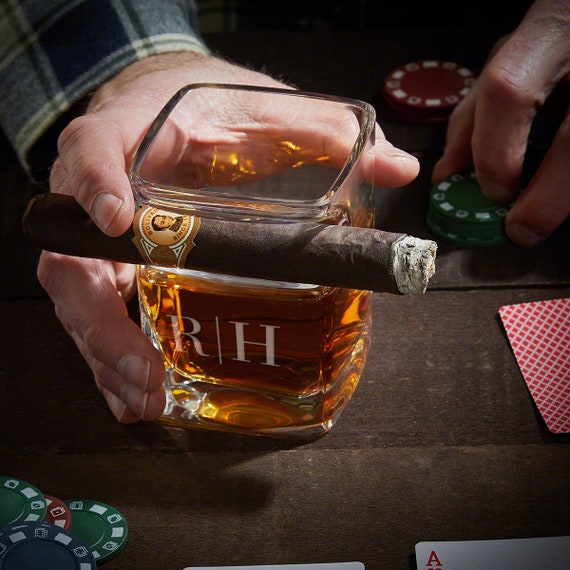In this photograph, a man, clad in a dark blue and light blue plaid long-sleeve shirt, is depicted in an intimate moment at a dark brown wooden table. His right hand, adorned with subtle lines and texture, elegantly grips a square glass filled with golden brown whiskey, the surface of the glass marked with the initials "RH" in white. Resting gently between his index and middle fingers is a lit cigar, its end adorned with a small gold emblem featuring a man's face. The glass also features an indentation specifically designed to hold the cigar. In his left hand, he clutches a stack of green poker chips, while additional stacks of red and green poker chips are scattered both behind and in front of the glass. Visible playing cards, including an ace of spades and a face-down card with a red and white checkered back, further emphasize the poker game setting. The wooden table's visible planks add a rustic charm to the scene, creating a detailed and evocative depiction of a classic, contemplative moment.